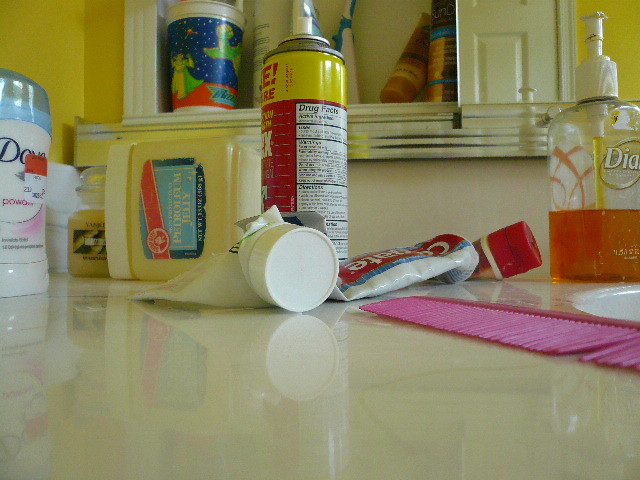A detailed glimpse into a bathroom sink countertop reveals a variety of everyday essentials neatly arranged. To the right, the edge of a porcelain sink is visible. Positioned above the sink is a half-full bottle of Dial soap, filled with vibrant orange liquid and featuring a pump handle. Immediately adjacent is a tube of Colgate toothpaste, recognizable by its distinctive red lid and red writing, flanked by a stripe running across its body. 

Lower in the frame, a pink comb rests on the marble-patterned countertop, adding a pop of color. At the center of the arrangement, a dual-colored hairspray bottle stands, transitioning from red at the base to yellow at the top. To its left, a jar of Vaseline lies on its side, and further left, a stick of Dove women's deodorant is placed, distinguished by its white packaging and light blue cap.

The backdrop of this organized chaos is a partially opened medicine cabinet, revealing a blue and green cup among other typical bathroom items. The marble design of the countertop ties the scene together, exuding both elegance and routine practicality.